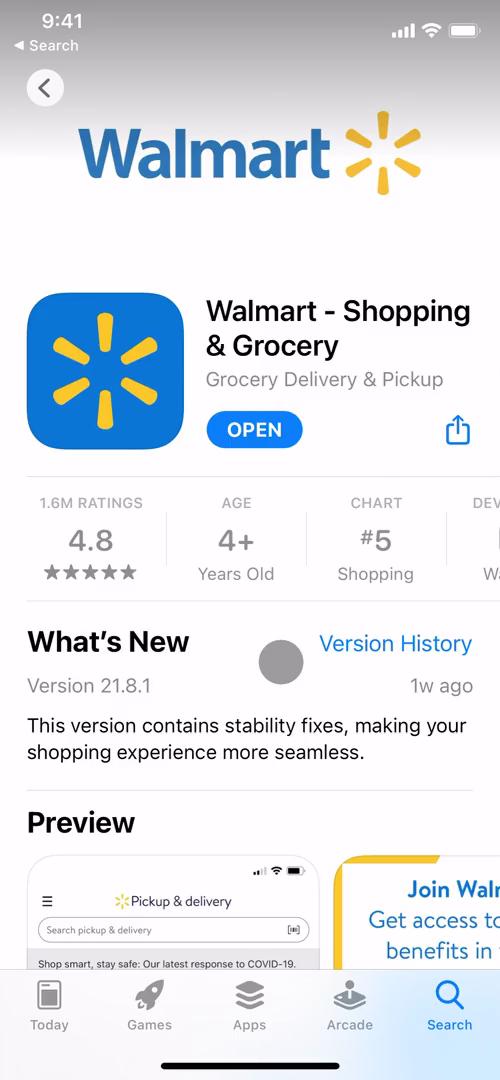This screenshot captures the display of the Walmart app on the App Store, viewed from a mobile phone. At the top, the brand name 'Walmart' is prominently displayed in blue text, accompanied by the recognizable yellow sunburst logo. The app's icon, a blue square with the same yellow sunburst logo, is prominently featured on the left side of the page.

Adjacent to the icon, the app's name 'Walmart - Shopping & Grocery' is printed in bold black letters. Below the name, a blue button labeled 'OPEN' invites users to launch the application. Further down, a gray section provides critical app details: it has garnered 1.6 million ratings, boasts an impressive average rating of 4.8 stars, is suitable for ages 4 and up, and ranks number 5 in the shopping category.

Beneath these statistics, sections titled 'What’s New' and 'Preview' offer additional context, with the latter displaying a couple of in-app screenshots to give potential users a glimpse of the app's interface and features. The bottom of this App Store page features a search bar alongside menus to navigate through different sections of the App Store.